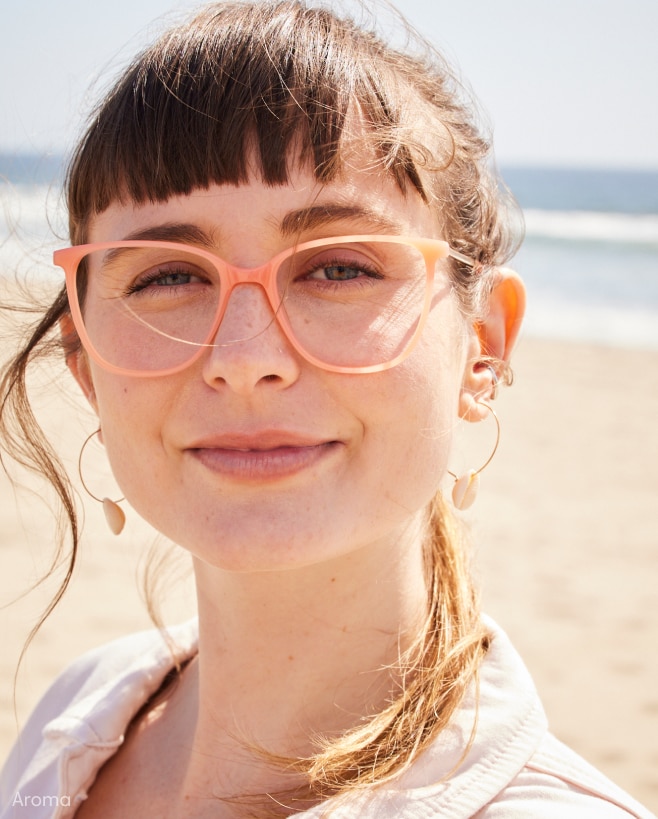This vibrant color photograph captures a young woman with a bright smile, centered and looking directly at the camera. Her brunette hair, adorned with bangs that end just above her eyebrows, flows down past her shoulders, with a few loose tendrils framing her face. She sports striking orange glasses that enhance her light blue eyes. Tiny freckles dot her fair skin across her face and neck. Her ears are decorated with large hoop earrings featuring seashell charms, adding a coastal flair to her look. She wears a blouse that appears to be a pinkish-white hue, reflecting the sunny ambiance. The backdrop showcases a picturesque beach with the ocean line visible, hinting at crashing waves and a bright sunny day. The bottom left corner of the image has the word "Aroma" prominently displayed in white letters.